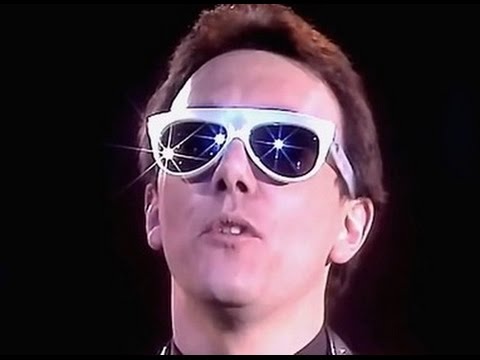The image captures a professionally taken still or video screenshot, likely from a music video or commercial dating back to the 1980s or 1990s. It features a Caucasian male, potentially a well-known musician or artist, with short brown or reddish hair, wearing distinctive white-framed sunglasses with thick rims, especially pronounced on the top. The lenses are very dark, perhaps black or dark blue, and within them, multiple lights are reflected, resembling small stars or suns. The man is looking off into the distance with a serious expression, his thin nose and slightly open mouth revealing a glimpse of his teeth. Though most of his clothing is obscured, he appears to be wearing a dark leather jacket or black fabric clothing. The background is a solid, deep black, making the focused, center-aligned image of the man stark and dramatic.